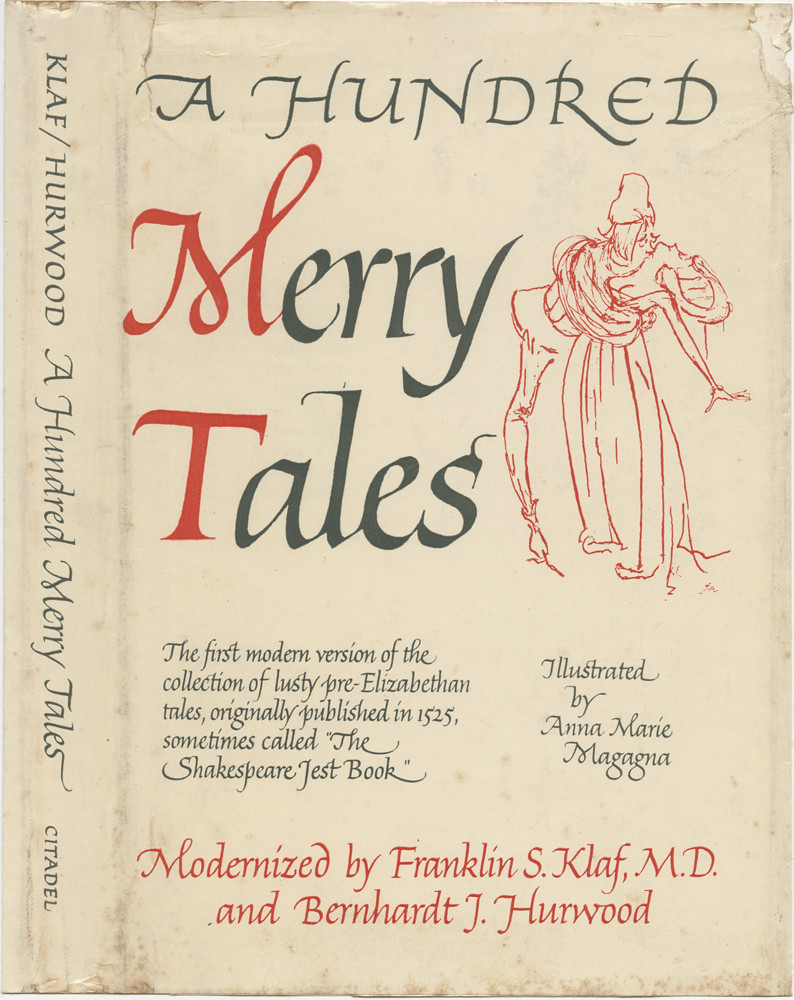The image depicts the cover and spine of an old, worn book titled "A Hundred Merry Tales." The cover features a beige background with the title prominently displayed. At the top in all caps and black letters is the word "A HUNDRED." Below it, aligned to the left, are the words "MERRY" and "TALES" stacked on top of one another, with the "M" and "T" in red and the remaining letters in black. A red and white line drawing of a woman in a fluffy dress, hands outstretched, is centered below the title. 

In smaller black text towards the middle-lower portion of the cover, it reads, “The first modern version of the collection of lusty pre-Elizabethan tales, originally published in 1525, sometimes called the Shakespeare Jest Book.” To the right of this text, it states, “Illustrated by Anna Marie Magagna." At the bottom, centered in red text, it says, "Modernized by Franklin S. Klaf, M.D., and Bernhardt J. Herwood." 

The left side of the image shows the spine of the book, with text written vertically in green. It reads, "Klaf / Herwood, A Hundred Merry Tales, Citadel," indicating the authors and the publisher. The overall appearance suggests the book is quite old and has been through significant wear and tear over the years.